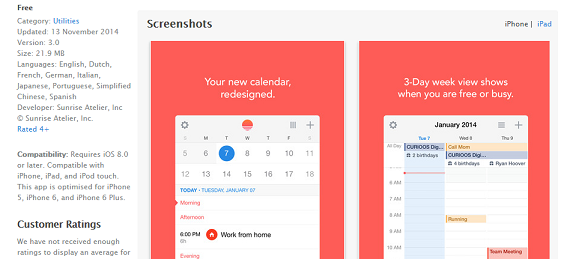The image prominently features a largely monochromatic palette with accents of red, primarily white and gray tones dominating the composition. In the top left corner, black text is displayed against a white background. The text reads, "Free Category Utilities Updated November 13, 2014. Compatibility requires iOS 8.0 or later. Compatible with iPhone, iPad, and iPod Touch. This app is optimized for iPhone 5, iPhone 6, and iPhone 6 Plus."

The central and right portions of the image showcase a gray background adorned with two red rectangular boxes. Each box contains white screenshots displaying various features of a calendar application. The two-thirds of the image to the right are dedicated to these visual depictions. The black text to the left remains legible, offering pertinent information about the app.

Within the first red rectangle located towards the center-right, bold white text announces, "Your New Calendar Redesigned." The second red rectangle, situated further to the right, contains text that reads, "Three-Day Week View Shows When You Are Free or Busy." This caption further suggests that the app in focus is a modern calendar tool designed to help users manage their schedules effectively.

Beneath the descriptive text in the left corner, there is a segment for customer ratings, although it appears incomplete and cut off, thus further details are not visible. Overall, the image seems to be an advertisement or an informational graphic for a calendar app, highlighting its redesigned interface and specific features tailored for older models of the iPhone.